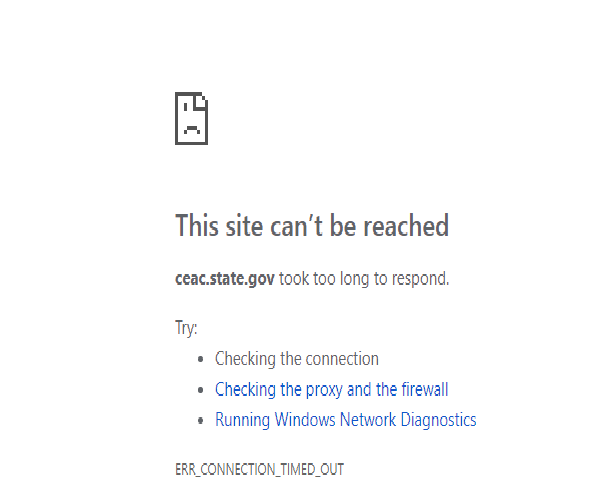A screenshot captures the familiar error message displayed when a website fails to load. At the top left corner, there is a small icon resembling a file with its top-right corner folded down, featuring an eye and a frowning face, symbolizing an issue or error. Below the icon, the message reads, "This site can't be reached." The specific site mentioned is "CAC.state.gov" which took too long to respond. The suggested troubleshooting steps include checking the connection, checking the proxy and firewall settings, and running Windows Network Diagnostics. The error code provided at the bottom is "ERR_CONNECTION_TIMED_OUT" with underscores separating the words.